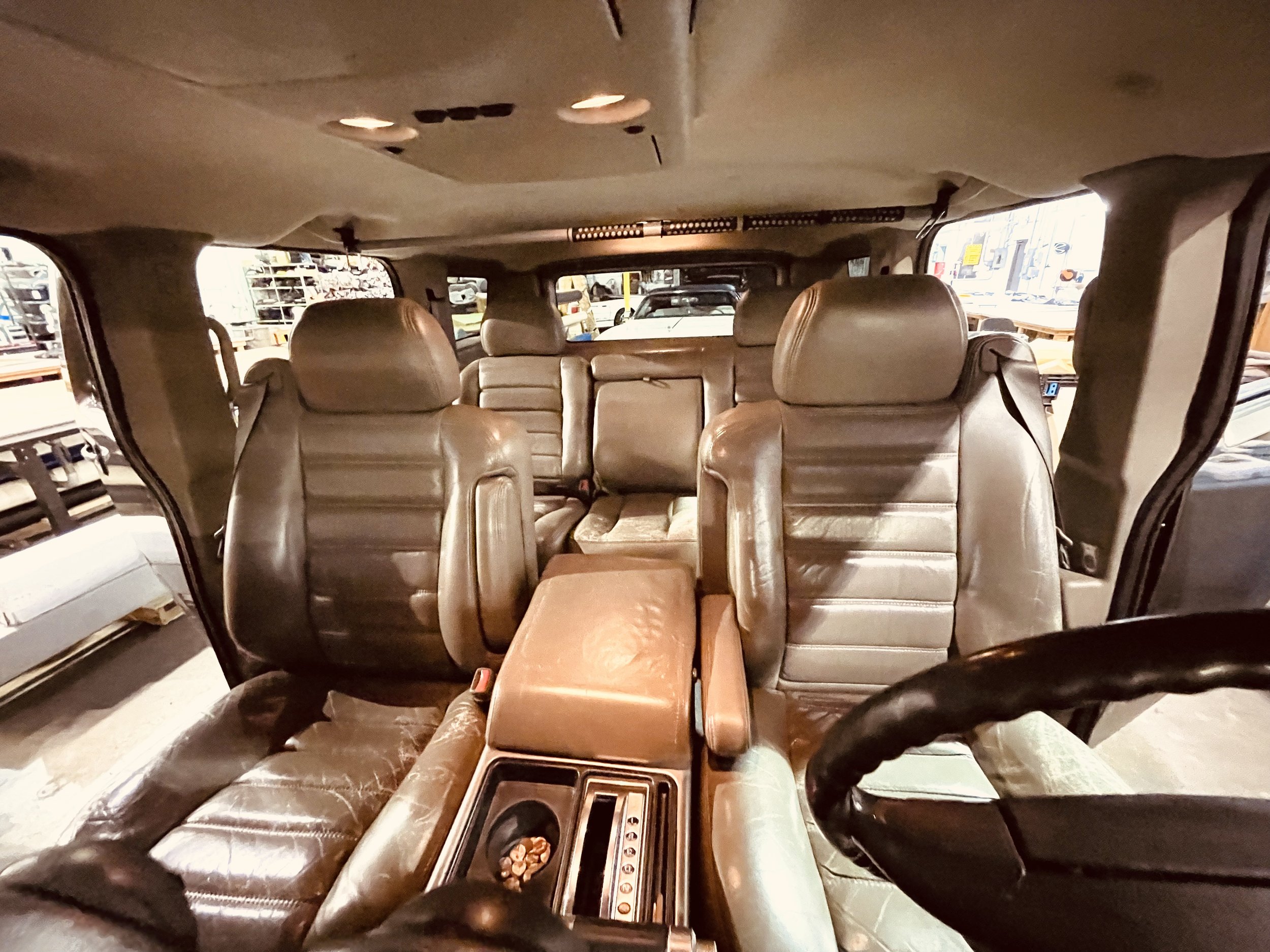The image reveals the spacious interior of an older car with an inviting, light brown and beige color scheme. The car’s front features two large leather-like seats, and the rear includes a matching bench seat comfortably seating three. Between the front seats sits a wide tan console, equipped with a gear shifter and a cup holder filled with what might be coins or small items. The brown steering wheel appears prominently on the right-hand side of the image, emerging from the lower corner. The absence of visible doors suggests they may be open or missing, providing clear views of the outside environment, including other cars and indistinct structures. The car's roof is illustrated in a cream color, complemented by three illuminated lights. The overall layout suggests a well-used, possibly vintage vehicle, with a cozy yet functional interior space.